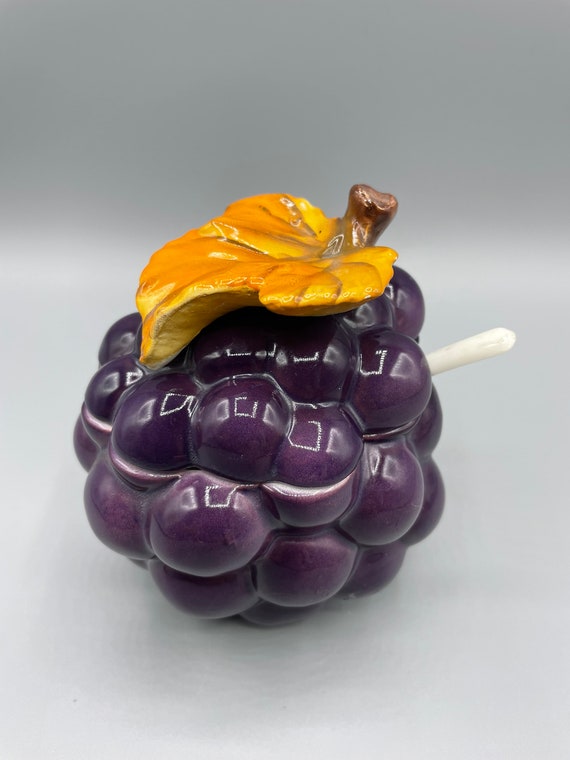The image features a highly detailed and glossy ceramic art piece designed to resemble a bunch of grapes. The grapes are a vibrant purple, presenting a shiny, reflective surface indicative of multiple layers of shellac. Each grape forms a bulb attached to a central stem. At the top of this grape bundle, there is an intricate ceramic leaf, painted in shades of orange and yellow, which is also glossy and reflective. On the side of the grape bunch, a white spoon is inserted, suggesting that this ceramic piece might double as a jelly or sugar container. The container appears to be split into a top and bottom section, with the spoon angled from the right side. The entire object rests on a light gray surface with a darker gray background, accentuating its colors and glossy finish.